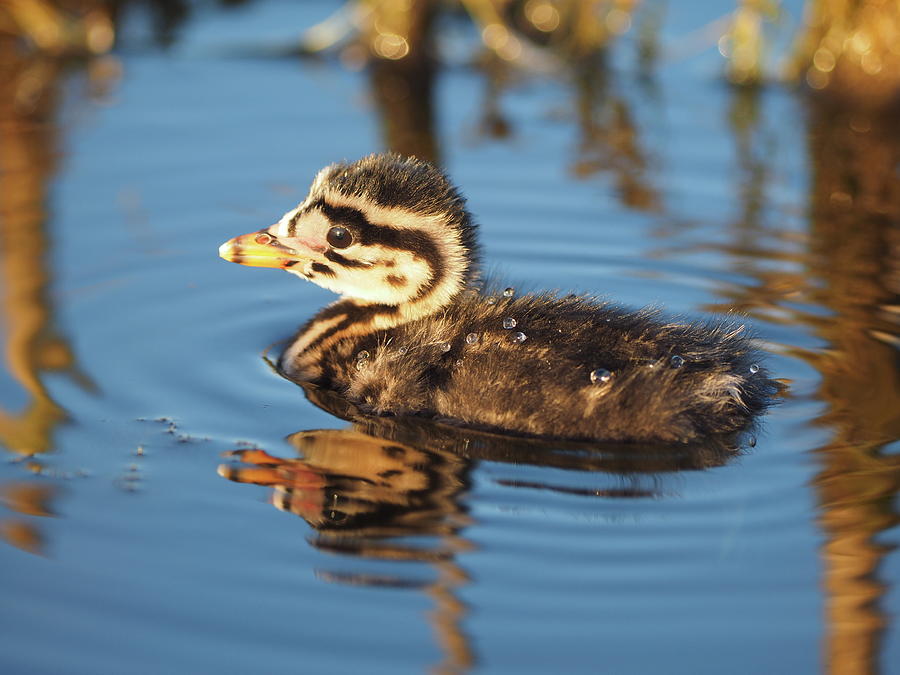This photograph features a baby duck, still in its infant stage, paddling serenely in the water. The little bird is solitary, with no other ducks nearby, as it glides through the water with small ripples and droplets on its back. The duck has a distinctive white face accented with dark lines around its eye, giving it a striking appearance. The top of its head is black, transitioning into a dark and light brown mix down its back, while its chest is adorned with white feathers. Its yellowish beak, tipped with a brown stripe at the end, adds to its charm. The water reflects the duck's head and body, creating a mirror image amidst the wavy ripples. In the background, reeds or other aquatic plants pierce the water's surface, adding a natural element to the scene.